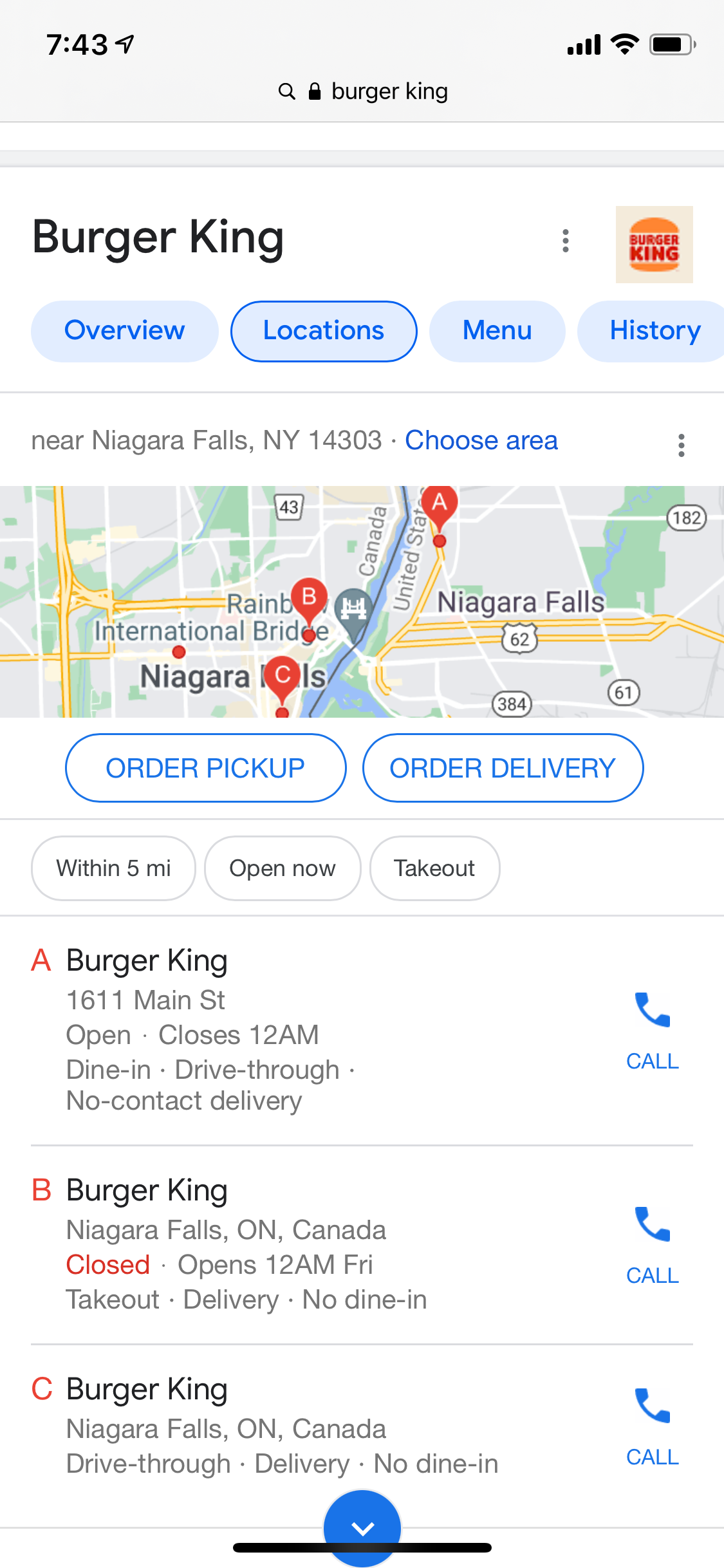This is a detailed, cleaned-up caption for the given image:

---

The image is a screenshot of a Google search for "Burger King" on a mobile app. At the top of the screen, the search bar displays "Burger King." Below the search bar, the header section with a white background prominently features the text "Burger King" on the top-left corner. Underneath the header, several categories are listed vertically.

Towards the bottom of the screen, there are navigational tabs labeled "Overview," "Locations," "Menu," and "History." Spanning the central portion of the screen is a wide map of New York City. The map is marked with three letters: A, B, and C, indicating the locations of different Burger King outlets. Each letter corresponds to red pin drops on the map, representing the specific positions of these Burger Kings.

In the middle of the bottom section, there is a blue circle with a downward-facing arrow, which can presumably be used to reveal additional information. Additionally, there is a thin black line spanning horizontally below the map, representing a carousel that allows users to scroll left and right through various images associated with the search.